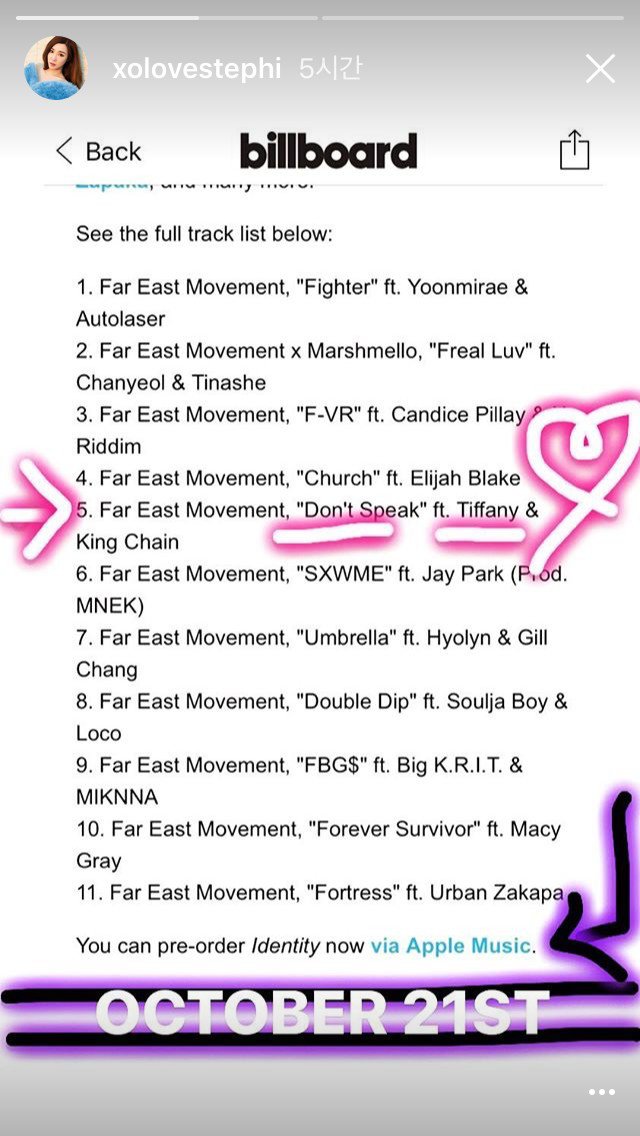This image appears to be a screenshot of an Instagram Story from the account 'xolovstephi.' The usual Instagram Story interface is visible, including the progress bar at the top indicating the current story segment being viewed. The profile name 'xolovstephi' is displayed prominently alongside a profile picture featuring an Asian woman. 

The content of the story is a screenshot, likely from a Billboard music chart, highlighting the tracklist of songs by Far East Movement. The list features 11 songs in total, with titles and featured artists specified for each. The tracklist includes:

1. "Fighter" by Far East Movement featuring Yumi De and Autolaser
2. "Free Your Love" by Far East Movement x Marshmello featuring Chanyeol and Tinashe
3. "Rhythm" by Far East Movement featuring FVR and Candice Pillay
4. "Church" by Far East Movement featuring Elijah Blake
5. "Don't Speak" by Far East Movement featuring Tiffany and King Chain

The fifth song, "Don't Speak," is particularly emphasized. It has been annotated with an arrow on the left margin, underlined, and a heart has been drawn next to Tiffany's name. This suggests a special fondness or personal connection to the song or the artist. 

At the very bottom of the list, the date 'October 21st' is noted, likely indicating when the chart was relevant or when the screenshot was taken. Moreover, the Korean text '시간' next to the profile name suggests it translates to 'hours,' perhaps indicating the time elapsed since the story was posted.